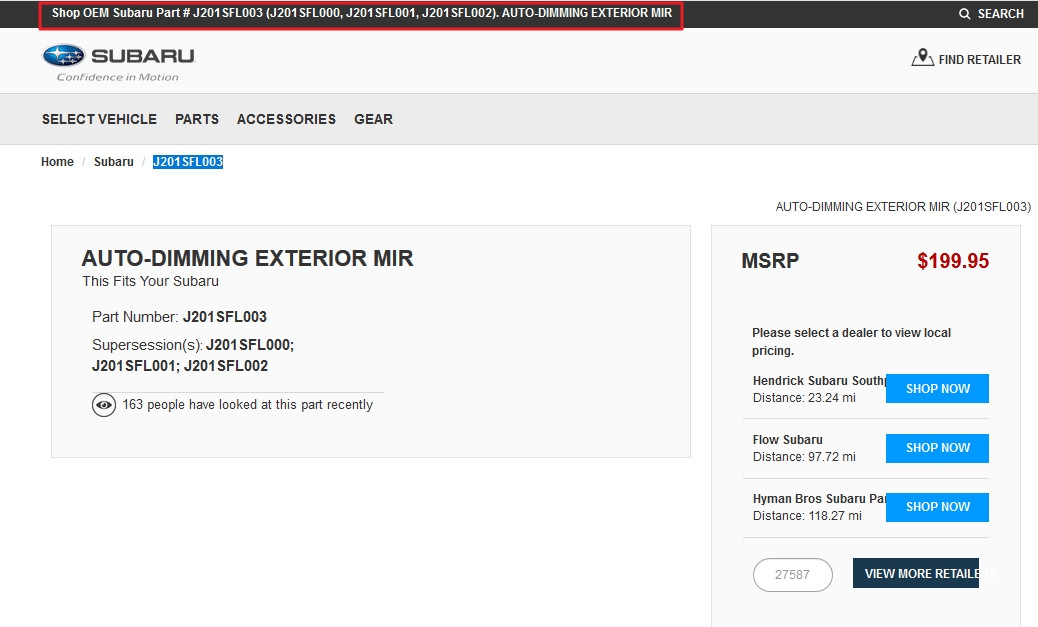### Descriptive Caption

The image is a detailed screenshot of a car modifier's website, specifically showcasing OEM Subaru parts for auto dimming exterior mirrors. It features a series of structured sections with clear typography, organized by headers, and sub-sections for easy navigation.

#### Top Header
The top header has a dark grey background with white text that reads, "Shop OEM Subaru Part Number J201SFL003, J201SFL000, J201SFL001, J201SFL002 Auto Dimming Exterior MIR," surrounded by a red border. On the right side of this header, there is a white search button accompanied by a search icon.

#### Secondary Header
Beneath the top header is a white header bar displaying the Subaru logo. To the right, there is a button labeled "Find Retailer" accompanied by a map icon. The white space between these elements is noticeable, likely for layout simplicity.

#### Navigation Bar
Below the secondary header, a grey background bar presents navigation options in dark text: "Select Vehicle," "Parts," "Accessories," and "Gear" on the left. The right side of this bar remains empty, highlighting the streamlined layout.

#### Breadcrumb Navigation
On a white background underneath, small text on the top left reads "Home, Subaru," with "J201SFL003" highlighted in blue, indicating the user's current navigation path. Adjacent is small text stating "Auto Dimming Exterior MIR, J201SFL003."

#### Main Content Section
The primary content area includes a rectangle with a light grey border on the bottom left. Inside, a white background presents black text reading "Auto Dimming Exterior MIR," with smaller text below stating, "This fits your Subaru." Below this, "Part Number" is displayed in bold text "J201SFL003," followed by "Super Sessions" listing J201SFL000, J201SFL001, J201SFL002. Beneath this list, a thin horizontal line separates the information from an eye icon, accompanied by the text "163 people have looked at this part recently."

#### Pricing Information
On the bottom right is another smaller rectangle with a light grey thin border. The title "MSRP" is at the top, followed by red text indicating "$199.95." Below this, centrally aligned black text reads "Please Select a Dealer to View Local Pricing" with a list of three different dealers, each with a blue "Shop" button beside them.

This comprehensive layout conveys essential information in a clear, structured format, optimizing the user experience for those seeking specific Subaru parts.